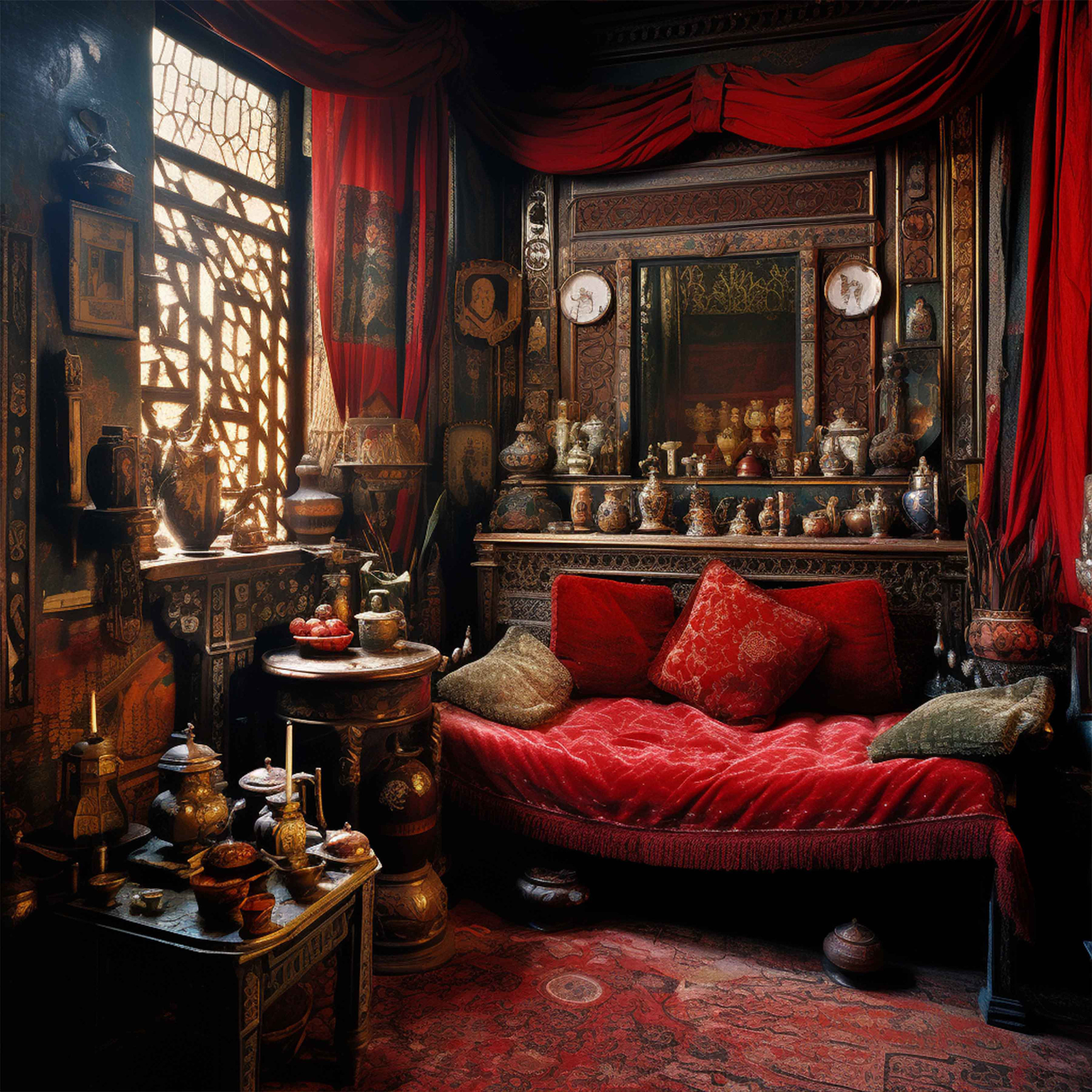The image depicts an Indian-themed room, rich in detail and antique charm. Dominating the room is a plush red sofa adorned with red velvet pillows and a couple of lighter-colored pillows, all set against what appears to be a decorated mantle or possibly a fireplace. Above the sofa hangs a mirror flanked by red horizontal curtains, with two shelves below holding an assortment of small jars and decorative items. The elaborate brown walls feature small shelves and are adorned with numerous vases and urns, accentuating the room's vintage atmosphere. On the bottom left, there is a small wooden stand cluttered with various items, and adjacent to the wall, a gold lattice-covered window allows sunlight to filter in, illuminating the rich, red, blue, and gray patterned rug on the floor. A short, rounded table, which holds a bowl of fruit, sits in front of the sofa. The room's thoughtful arrangement of antique wooden shelves and decorative elements creates a visually captivating and historically rich ambiance.